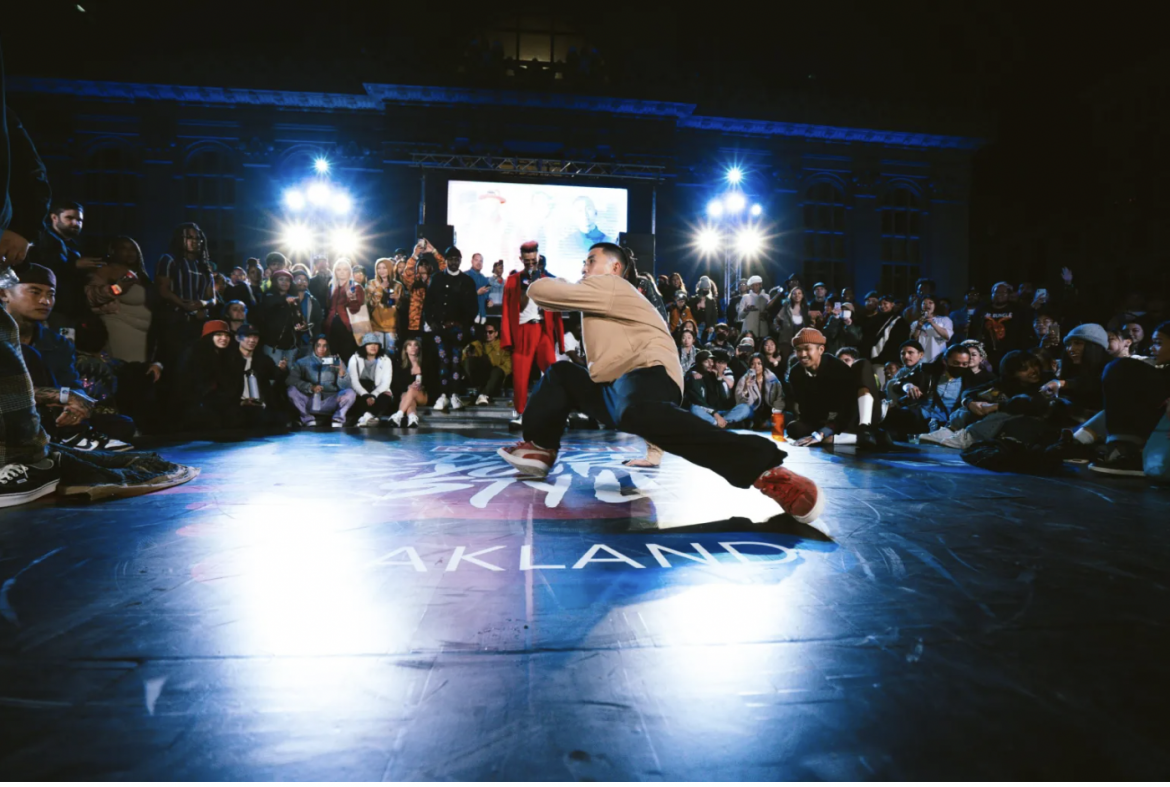In this nighttime outdoor photo, a person is break dancing on a stage-like mat with the word "Oakland" partially visible, faint due to the bright spotlights. The dancer is captured in an acrobatic pose, with one hand on the ground for support and the other arm raised, looking to the side, while their legs are spread apart. They are wearing a light tan jacket, black baggy pants, and red and white Puma sneakers. The image is taken from a low angle, almost ground level, highlighting the dancer’s dynamic movements. Surrounding the stage are several rows of spectators, with the closest rows sitting on the ground. In the background, behind the crowd and spotlights, there's the exterior of a large brick building with a projection screen. The floor they are dancing on appears to be a shiny, plasticky surface, likely set up specifically for the performance.